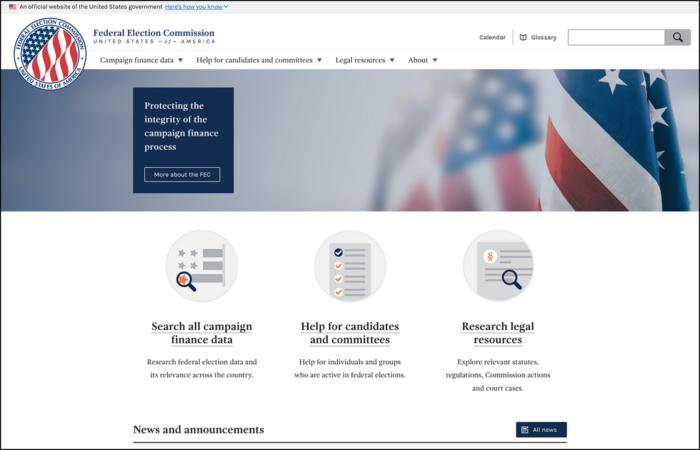This screenshot captures the homepage of the Federal Election Commission (FEC) website. At the very top, a horizontal gray bar spans the width of the page. In the upper left corner, there is a small American flag icon, followed by the text, "An official website of the United States government," in a readable font. To the right of this text, in blue lettering, it states, "Here's how you know," accompanied by a drop-down arrow.

Beneath this header, there is the official FEC logo on the left, featuring a flag-like design in the center. Adjacent to the logo, the words "Federal Election Commission, United States of America," are clearly displayed.

The navigation bar directly below includes several sections: "Calendar," "Glossary," a search bar, "Campaign Finance Data" with a drop-down menu, "Help for Candidates and Committees" with a drop-down menu, "Legal Resources" with a drop-down menu, and "About" also featuring a drop-down menu.

Occupying the upper third of the screenshot is a photograph of the American flag situated on the right side of the page. On the left side of this section, there is a prominent blue box containing the text, "Protecting the Integrity of the Campaign Finance Process," followed by a link that reads, "More about the FEC."